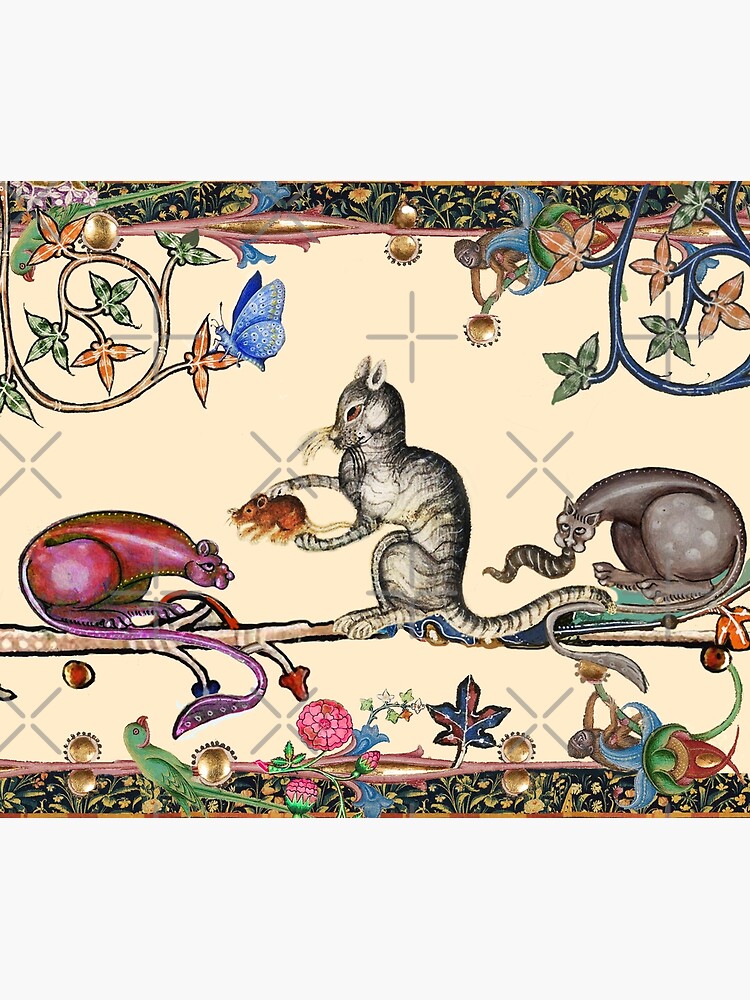The painting features three cats in an ancient, pre-Renaissance style reminiscent of cave paintings. On the left, a pink cat is depicted, while in the center a gray cat holds a mouse in its mouth. To the right, a black cat is seen with a striped tail or snake emerging from its mouth. The image is bustling with an array of additional elements, including birds, butterflies, a green parrot, and flowering plants. Among the blooms, there is a curious detail of gorilla heads, seemingly part of the floral design. Scattered throughout the artwork are distinctive watermarks of plus signs and X's, giving it a crosshatch effect. Golden balls are interspersed within the composition, and banners adorned with flowers frame the top and bottom of the scene, adding to the intricate and abstract nature of the painting.